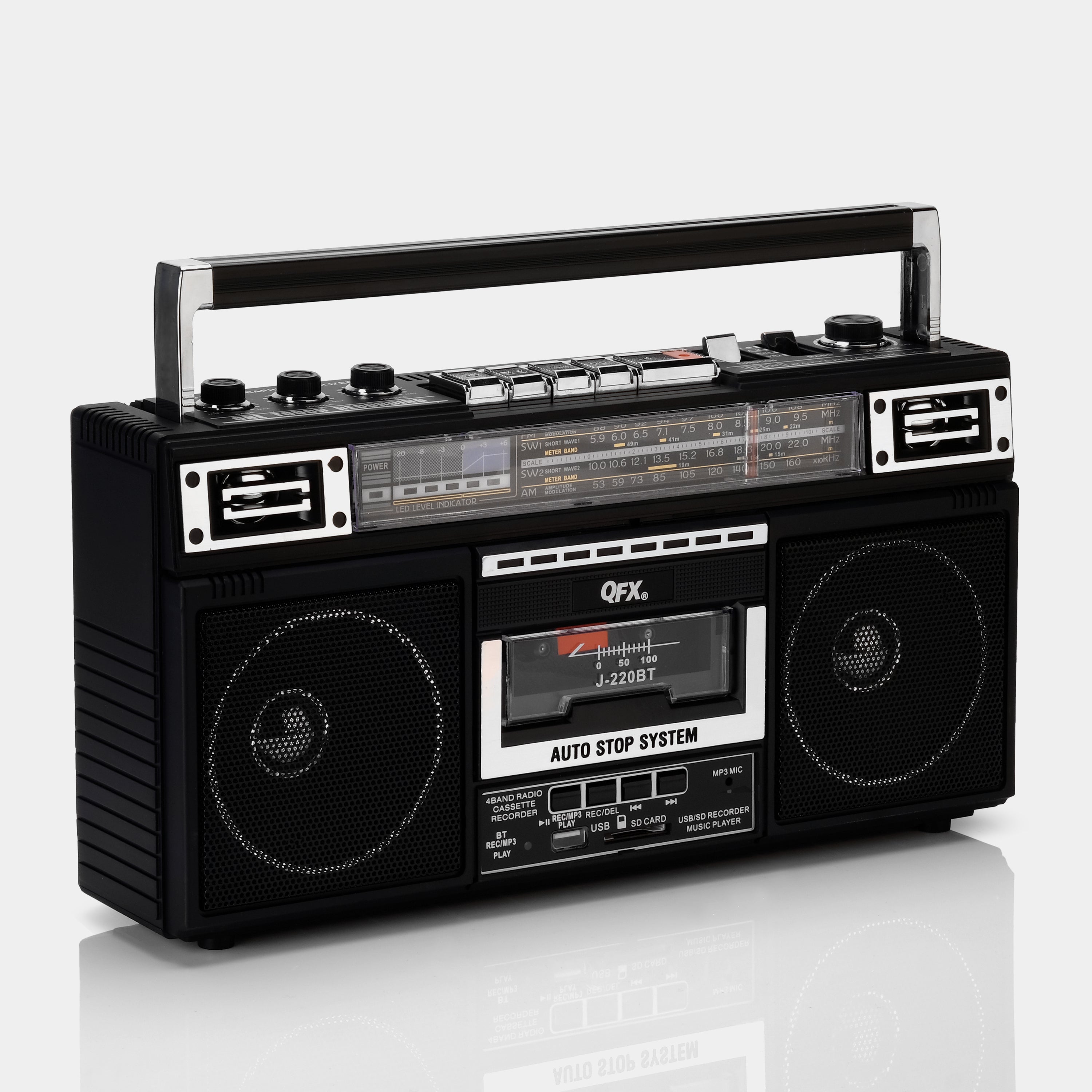This image depicts an old-school black QFX boom box, viewed from the front and slightly angled to the left. The boom box features two prominently outlined speakers on either side of a central cassette tape player, adorned with a silver trim and a white banner that reads "auto stop system." Above the player, which identifies itself as the model "J-220BT," is a QFX logo. Below the cassette deck are buttons for functions such as fast forward, rewind, and play. The device's top panel includes various controls: three knobs on the left for adjusting bass, treble, and volume, five silver buttons (four smaller and one larger), a yellow toggle switch, and another round black knob on the far right. The handle, designed for portability, is straight up with silver sides and a black grip.